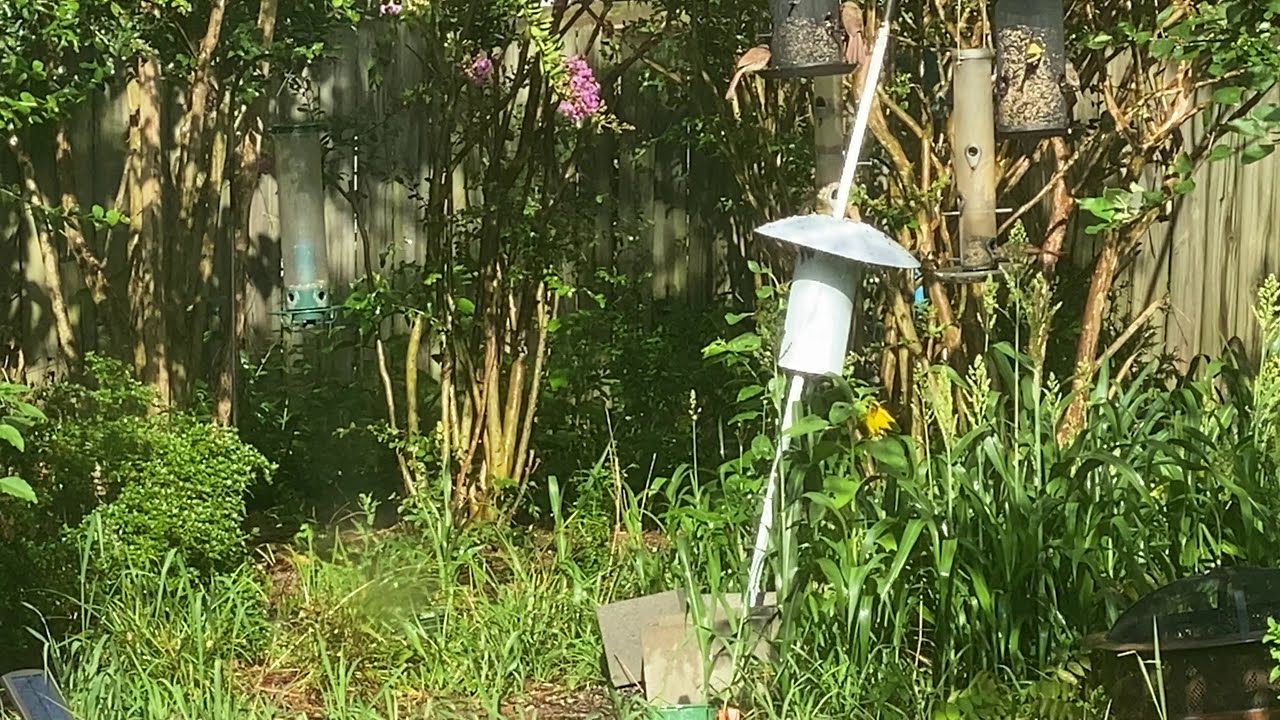The image depicts an overgrown backyard garden bordered by a weathered gray wooden fence. Several bushes, possibly including lilac bushes with purple flowers, populate the area, interspersed with tall, lanky grass and weeds. Among the greenery, numerous bird feeders are visible; two are in the distance on the right, each visited by birds, and another white feeder on a tilted metal pole stands prominently in the foreground, reflecting light brightly. Additionally, two bird feeders are hanging on the right, one of which is tinged blue. A patch of yellow wildflowers grows near the right corner, mingling with the overgrown grass. Notable ground features include scattered concrete blocks and the top of a fire pit in the lower right corner. The scene captures a densely vegetated, somewhat wild garden with various elements that suggest a bustling, nature-friendly environment.